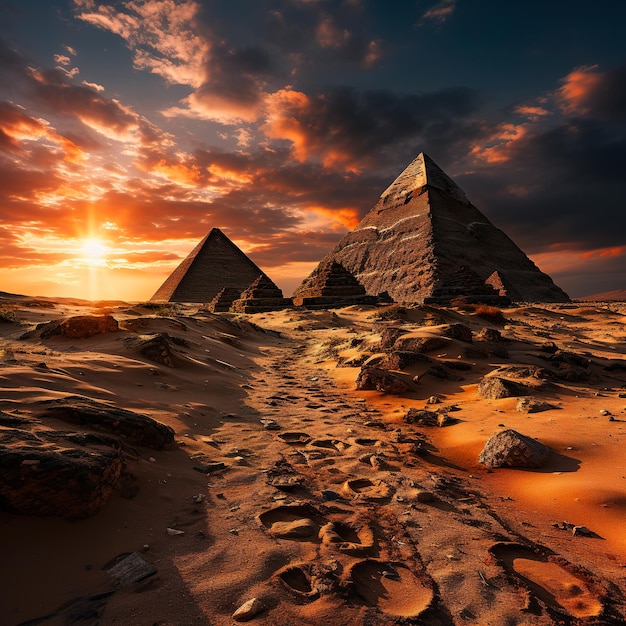This square, AI-generated image features a surreal landscape dominated by pyramids, seemingly situated on another planet. The composition places a large pyramid slightly towards the right of the frame, with a smaller pyramid in the background to the left and three diminutive, rough-textured pyramids in the foreground. The terrain, reminiscent of a desert, has a lunar-like quality with its rocky, uneven surface. The coloring of the scene is predominantly in darkish browns and oranges, likely enhanced by a filter. This color palette is further dramatized by the rising or setting sun in the background on the left-hand side, casting a bright light that illuminates the sky filled with orange-tinged clouds against a dark blue backdrop. Footprints can be seen leading through the sand, adding to the sense of a mysterious journey through this otherworldly landscape.